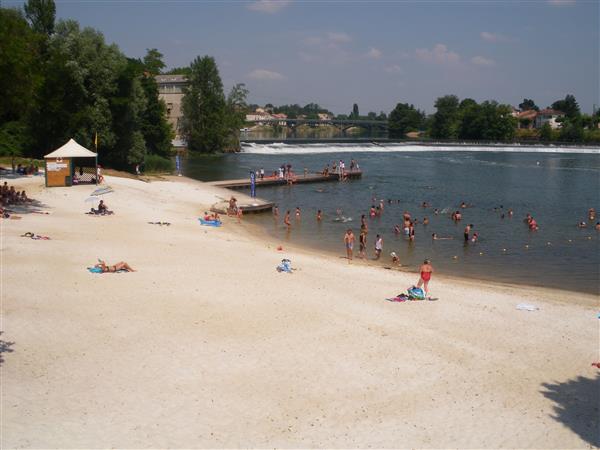This image depicts a lively beach scene by a lake, framed from a distance. The sandy shore is light brown and well-maintained, suggesting a family-friendly and clean environment, with no visible signs of trash. A variety of people occupy the area; some are laying on towels soaking up the sun while others are in the blue water, enjoying a swim. In the foreground, there's a woman in an orange swimsuit, and about three or four people laying out on towels. The beach is dotted with pine-like trees, further indicating a lakeside setting rather than an ocean.

A small wooden pier extends into the water where people are standing, adding to the scene's dynamic. To the left of the pier, there's a charming little hut that could possibly be a refreshment stand, distinguished by its white roof. Additionally, another small hut with a red cross sign suggests the presence of a lifeguard, ensuring safety for all the beachgoers.

In the background, nestled within greenery, are buildings that resemble a resort area, potentially hotels or homes, adding a touch of civilization to the natural setting. The image captures a warm, enjoyable day at the beach, filled with energy and relaxation.